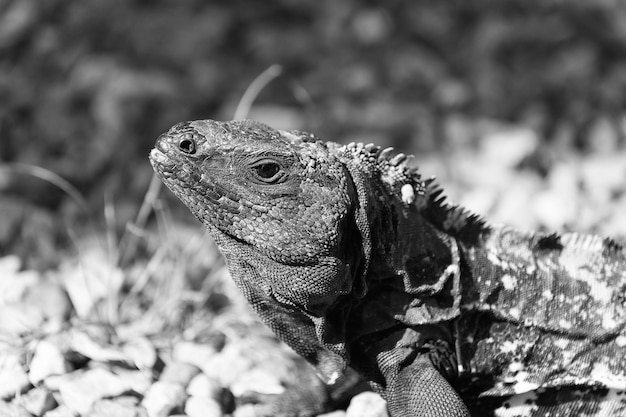In this detailed black-and-white photograph, an iguana is prominently showcased in its likely natural outdoor setting, surrounded by rocky terrain and a touch of grass. The iguana's head is positioned slightly left of center and appears to be looking upwards and to the left. The creature's head is adorned with intricate scales, clearly visible due to the close-up. Its nostrils are at the end of its snout, and a beady eye can be seen just behind. A defined ridge separates the head from the rest of the body, and spiky scales run along its back. The iguana's body stretches back and to the right, exiting the frame at the bottom right edge. Its legs are partially visible; the left leg can be seen more clearly compared to the right, which blends into the rocky ground. The iguana’s skin has a textured pattern with gray and white specks, complemented by a subtle checkered design on its legs. The background is out of focus but suggests the presence of grass and possible wooded vegetation, adding to the natural ambiance of the scene.